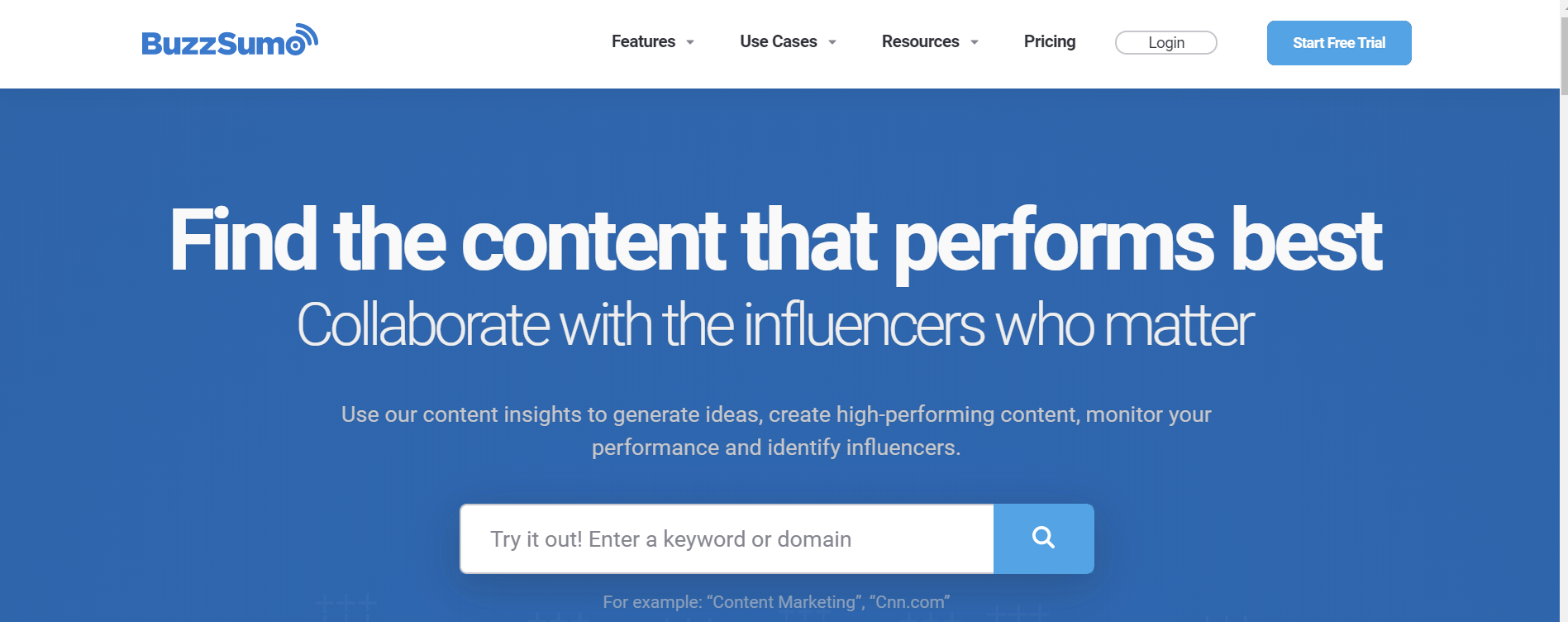This is a detailed screenshot of the BuzzSumo website. At the top left corner, the BuzzSumo logo is prominently displayed in blue text. Adjacent to it, a navigation menu occupies the upper section of the page against a white background, featuring black text options for 'Features,' 'Use Cases,' 'Resources,' and 'Pricing.' Additionally, there is a 'Login' button and a 'Start Free Trial' button in blue.

Beneath this navigation bar, a large blue banner commands attention with the bold text: "Find the content that performs best, collaborate with the influencers who matter." Just below this statement, it elaborates further: "Use our content insights to generate ideas, create high-performing content, monitor your performance, and identify influencers."

Following the banner, there is a search bar inviting users to "Try it out." Users are prompted to enter a keyword or domain, with suggestions like "content marketing" or "CNN.com" provided as examples. The search function is completed with a blue search icon.

The color scheme of the screenshot is limited to black, blue, and white, creating a clean and professional appearance.